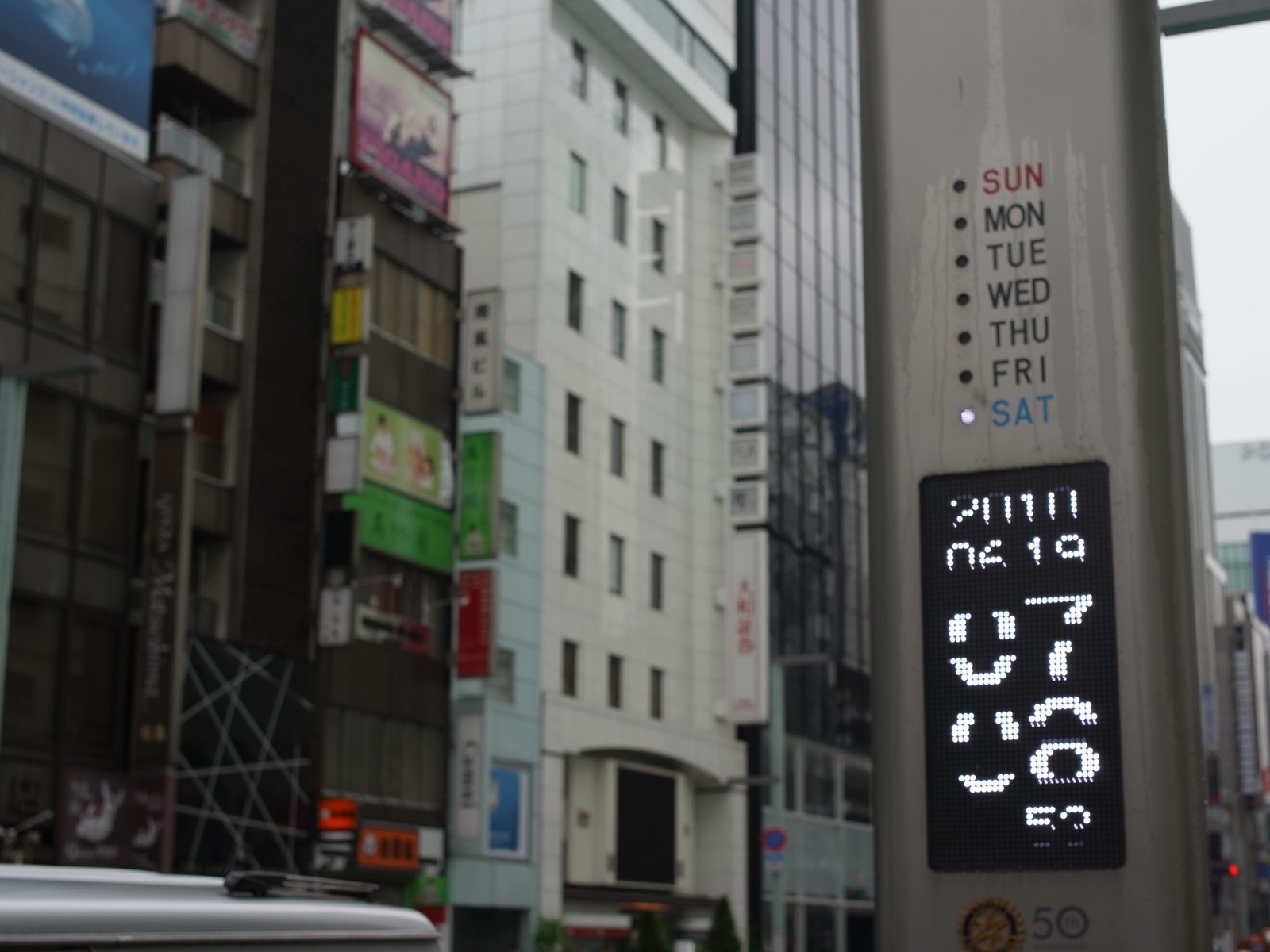This photograph captures a bustling cityscape, showcasing an array of towering structures, likely comprising office buildings and apartments. Dominating the left side of the image is a skyscraper adorned with numerous windows arranged in a grid-like pattern. Adjacent to this is a slightly shorter, white building, featuring fewer windows. Nearby, a collection of vibrant billboards stacked atop each other draws attention with a mix of green, pink, and red hues, contributing to the urban aesthetic.

On the right side, a distinctive pole catches the eye, serving as an informational display. The pole features a digital section showing the current day of the week, Saturday, highlighted in blue. Beneath this, a digital screen presents the current date and time, with white text against a black background. This detailed snapshot vividly encapsulates the dynamic and multifaceted character of city life.